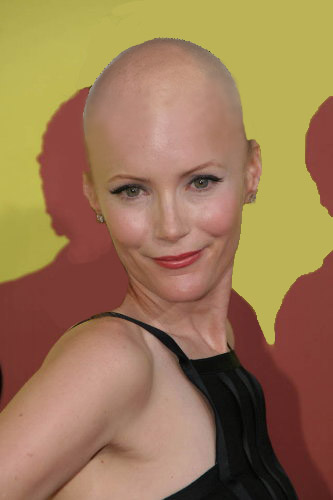This is a photograph of a fair-skinned woman with a bald head, who is likely wearing a bald cap. She is dressed in a thin-strapped black dress and has makeup including eyeliner, mascara, and red lipstick. The woman is positioned at the center of the image from the chest up, with her body angled sideways and her face turned towards the camera, offering a subtle smile. Behind her is a yellowish-green wall adorned with maroon and burnt-orange silhouettes of people. The overall style suggests a poised yet unique portrait, possibly artistic or editorial in nature.